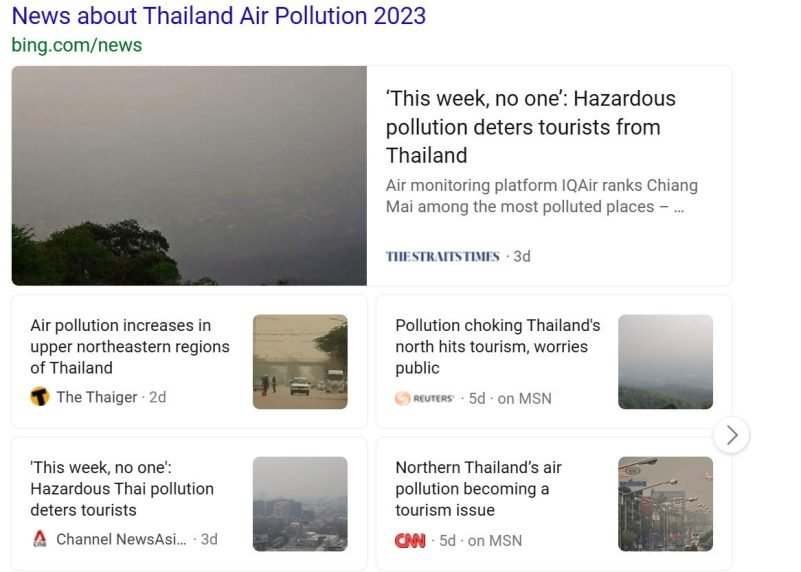**Detailed Image Caption:**

This screenshot captures a web page featuring news about Thailand's air pollution in 2023. At the top, the headline "News about Thailand air pollution 2023" is prominently highlighted in dark blue font. Directly below the headline, the source is identified as "bing.com/news."

The main image shows a dark gray sky with visible tree tops, illustrating the severity of air pollution in the region. To the right of this picture, a highlighted quote reads, "This week no one," referencing the hazardous pollution levels deterring tourists from visiting Thailand. The air monitoring platform, IQ Air, ranks Chiang Mai among the most polluted places. The source of this information appears to be "The Straits Times," dated three days ago.

Beneath the main image, there are four smaller images accompanied by article titles:

1. **Upper Left Image:** A street scene under a gray, foggy, or polluted sky, with a car and two people standing on the street. The title reads, "Air pollution increases upper northeast regions of Thailand," posted by The Thaiger.

2. **Upper Right Image:** A mountainous landscape with treetops visible under a gray, hazy sky. The title states, "Pollution choking Thailand's North hits tourism, worries public," reported by Reuters on MSN from five days ago.

3. **Bottom Left Image:** A cityscape under a gray, hazy sky. The title quotes, "This week no one," referring to the hazardous Thai pollution deterring tourists. This article is from Channel News Asia.

4. **Bottom Right Image:** Another city scene with a hazy gray sky, with the title, "Northern Thailand's air pollution becoming a tourism issue," posted by CNN.

The screenshot effectively portrays the widespread concern and coverage of Thailand's significant air pollution problem and its impact on tourism.